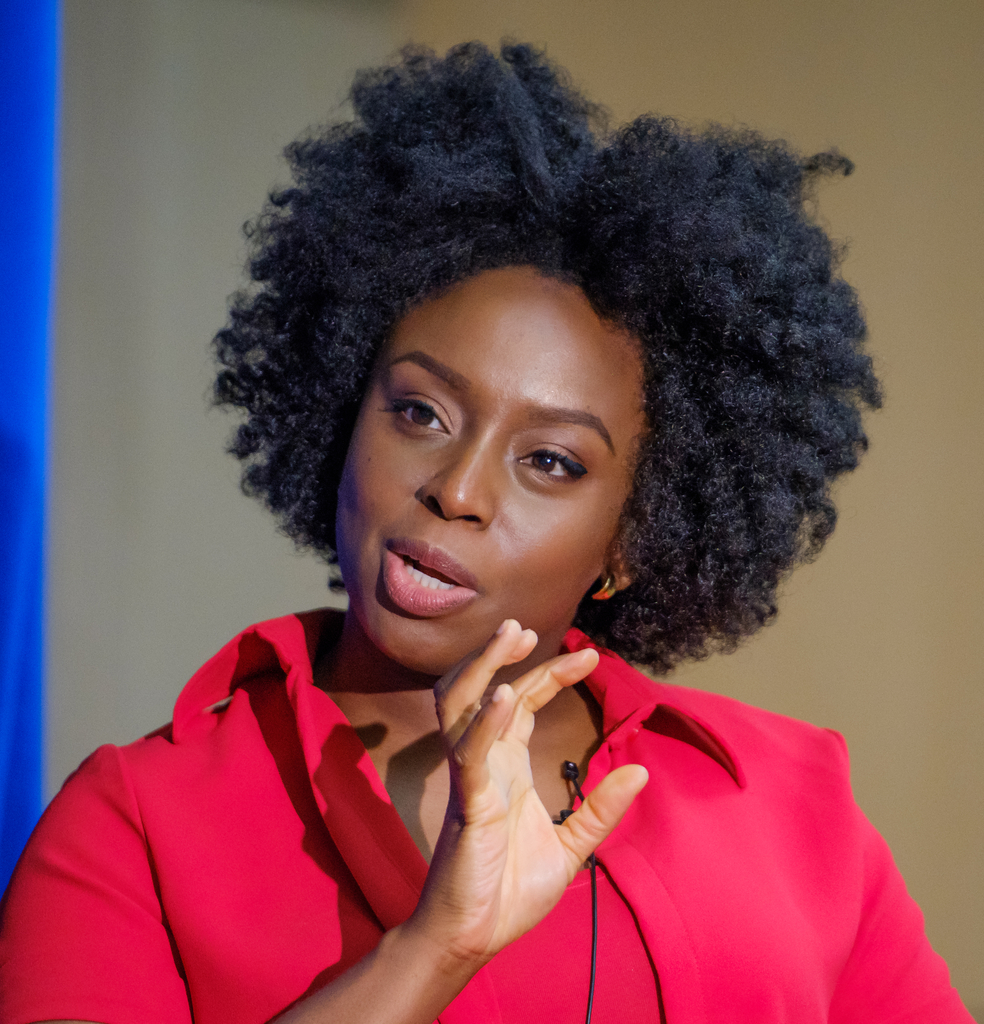The image captures a young Black woman with short, thick, curly hair, engaged in a conversation. She is depicted from the shoulders up, wearing a vibrant, shocking pink jacket with a collar over a top. A small black microphone is clipped to her jacket. She makes expressive gestures with her right hand, which is slightly open and raised. Her head is slightly tilted to the right, her mouth is slightly open revealing her teeth, and she wears a distinct earring shaped like an animal tooth, colored in golden and orange hues. The background features a grayish-brown wall with a blue vertical stripe or curtain on the left side.